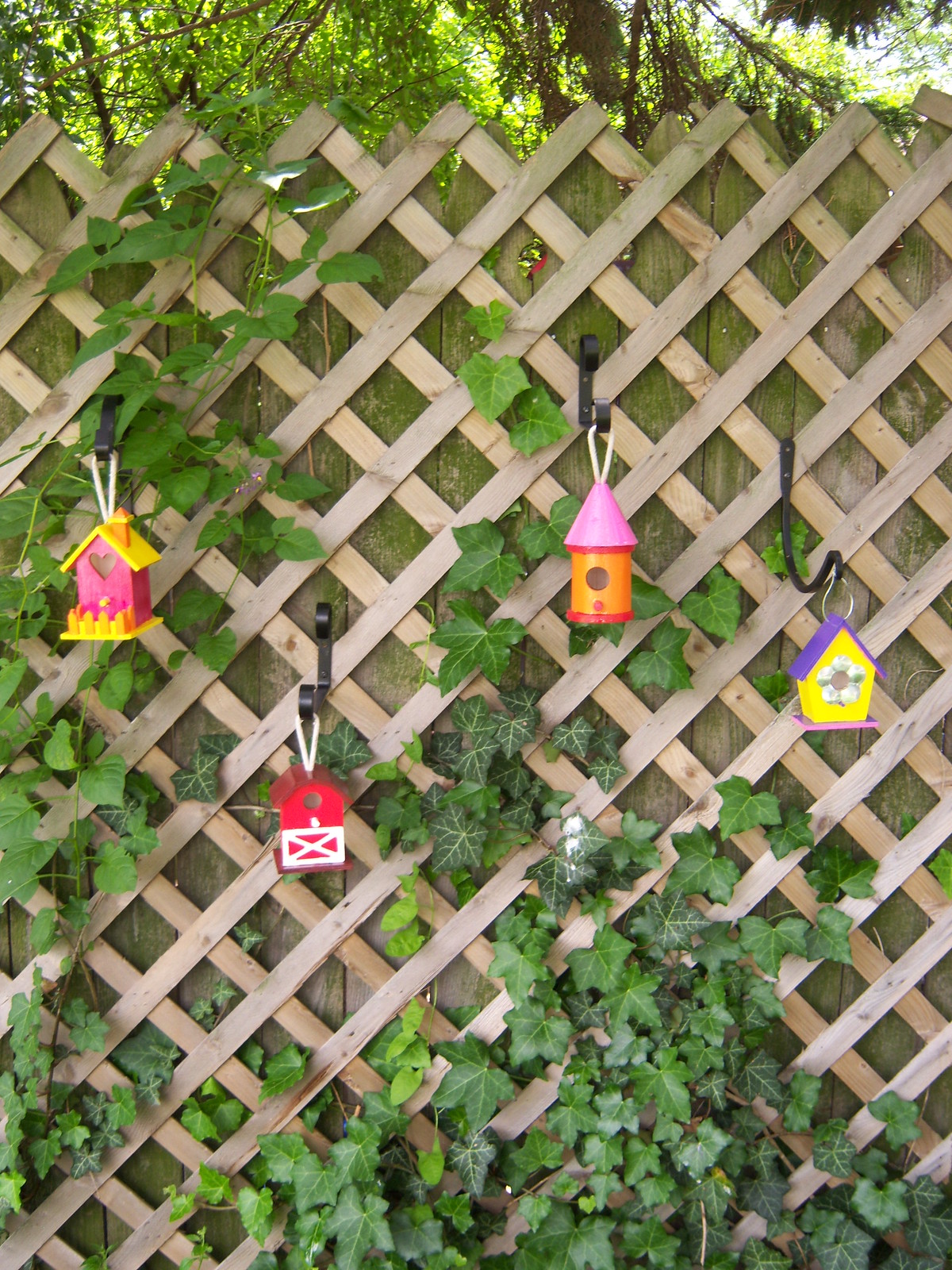This outdoor photograph showcases a tall wooden latticework fence, featuring a criss-cross design with a solid backing of straight wooden planks. The fence is adorned with climbing vines and is set against a backdrop of lush trees. Four colorful birdhouses hang from hooks on the fence. The first birdhouse is pink with a yellow roof, the second is red and white resembling a little barn, the third is orange with a pink cone-shaped top resembling a castle tower, and the fourth has a yellow body with a purple roof.